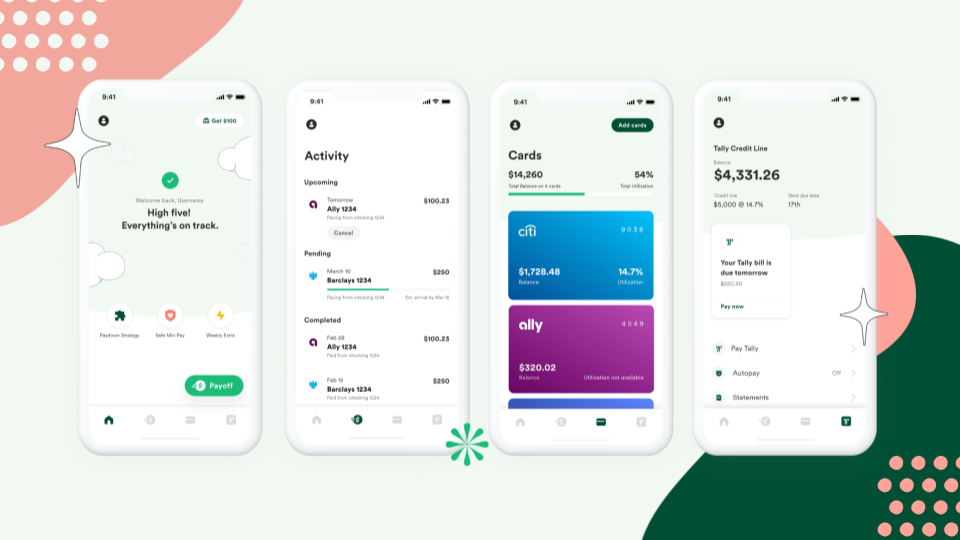This image displays a detailed presentation slide reminiscent of an advanced poster board, outlining what users can expect when utilizing a specific financial management app. The presentation is divided into four distinct slides, each representing a different feature or page within the app.

1. **First Slide:** The introductory page of the app greets the user with a positive affirmation, "High five! Everything's on track." While some settings are partially obscured, a prominent button labeled "Pay Off" indicates an option to manage debt or payments, suggesting that the app serves as a financial management tool, possibly like a mini wallet.

2. **Second Slide:** This section details the user's recent activity, showcasing transactions or payments that have been made. It likely provides a comprehensive summary of the financial actions taken by the user, aiding in tracking and reviewing past expenses.

3. **Third Slide:** Here, a list of available cards is displayed. The specific cards mentioned include the Citi Card and the Ally Card, indicating that the app allows users to manage multiple credit or debit cards in one place, enhancing convenience and organization.

4. **Fourth Slide:** The final segment presents an overview of the user's total credit line along with the respective amounts and upcoming bills. This slide is crucial for users to monitor their credit usage and ensure timely bill payments.

Overall, the presentation effectively communicates the app's capability to serve as a comprehensive financial management tool, helping users track their spending, manage multiple cards, and stay on top of their financial obligations.